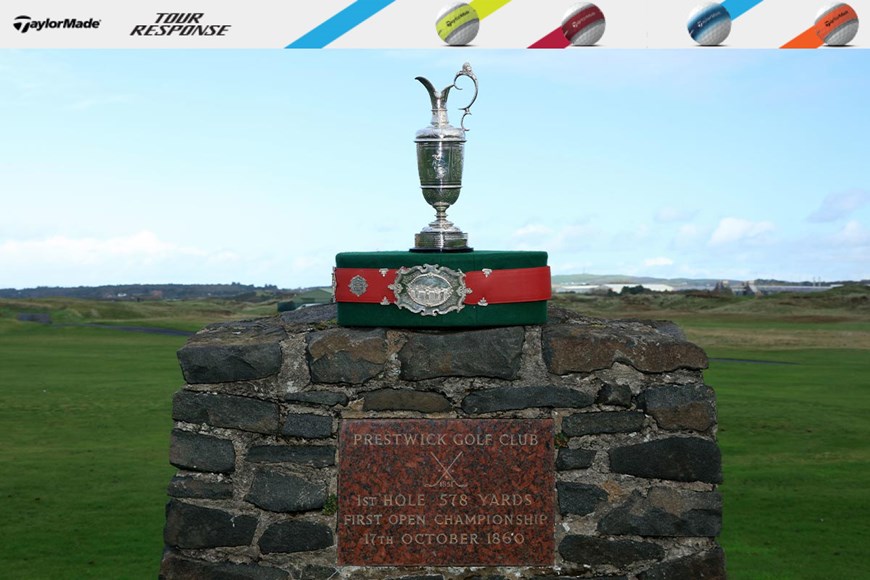In this outdoor photograph taken at a golf club, a silver trophy is prominently displayed atop a stone pedestal set in a lush, green pasture against a backdrop of clear blue skies. The trophy, resembling a chalice with an ornate handle on its right side, sits on a green base encircled by a red wrapped belt. In front of it is a silver plaque. The stone pedestal, part of a small built-up stone wall, features a red plaque that reads: "Prestwick Golf Club, first hole, 578 yards, first Open Championship, 17th October 1860," with two crossed golf clubs engraved above the text.

At the top of the image, a white banner showcases the TaylorMade logo and the text "Tour Response." The banner is adorned with five colorful sections—blue, yellow, red, blue, and orange—each featuring a TaylorMade golf ball with corresponding stripes. The vivid colors of the banner contrast with the serene greens and blues of the golf course, creating a vibrant, detailed composition.